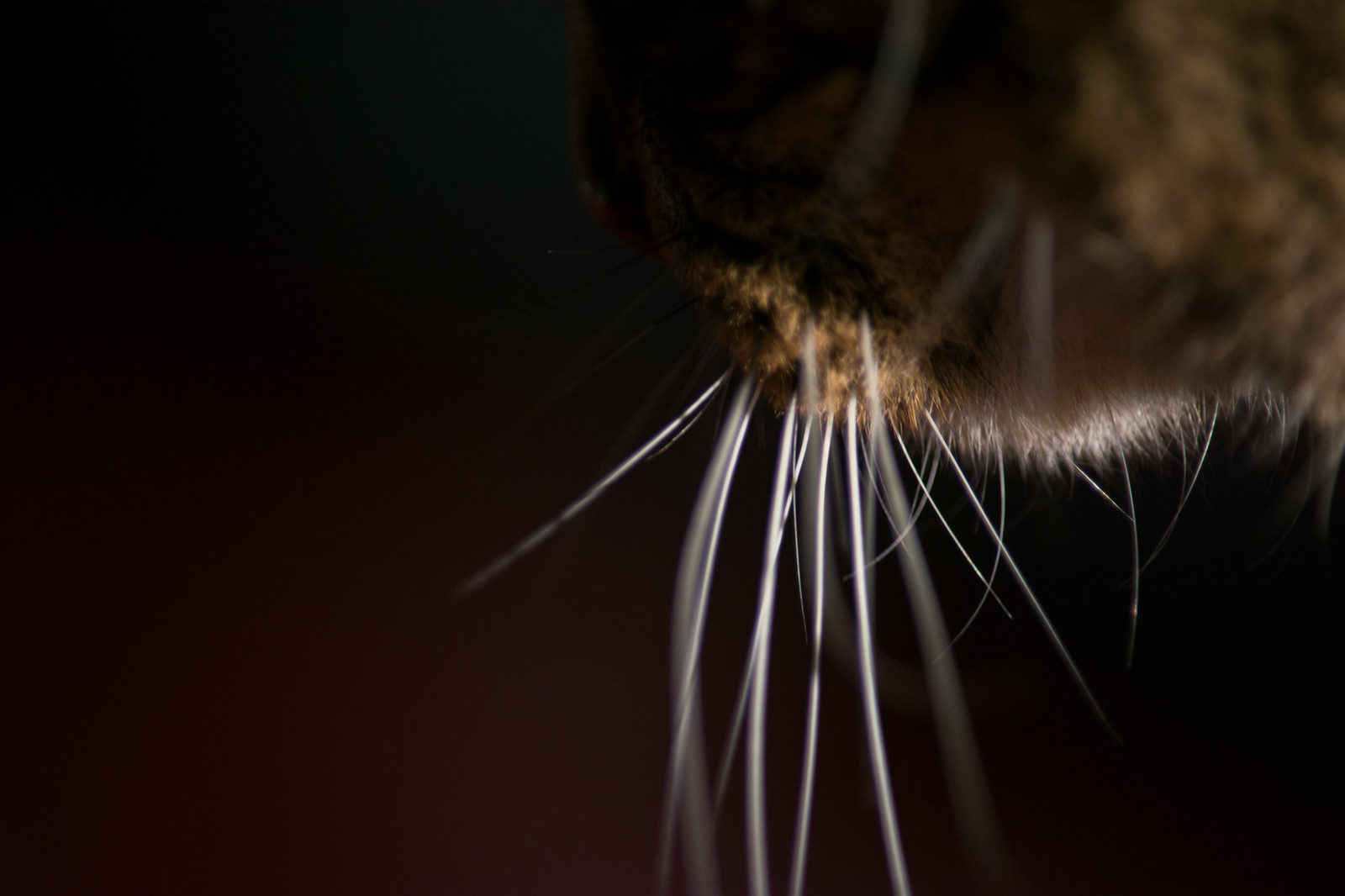This close-up color photograph captures the intricate details of a possibly nocturnal brown and black-furred mammal, heavily emphasizing its white whiskers. The animal's face occupies the top right corner of the image, its fur varying from dark brown to lighter shades beneath its chin. Illuminated by a flash or a light source from below, the white whiskers glow conspicuously against the dark background, which transitions from a dark burgundy at the bottom to pure black at the top. The photograph, taken in landscape orientation, showcases the animal against the solid, undisturbed backdrop, highlighting the coarse texture of its short fur and the prominent, protruding whiskers extending toward the center of the image.